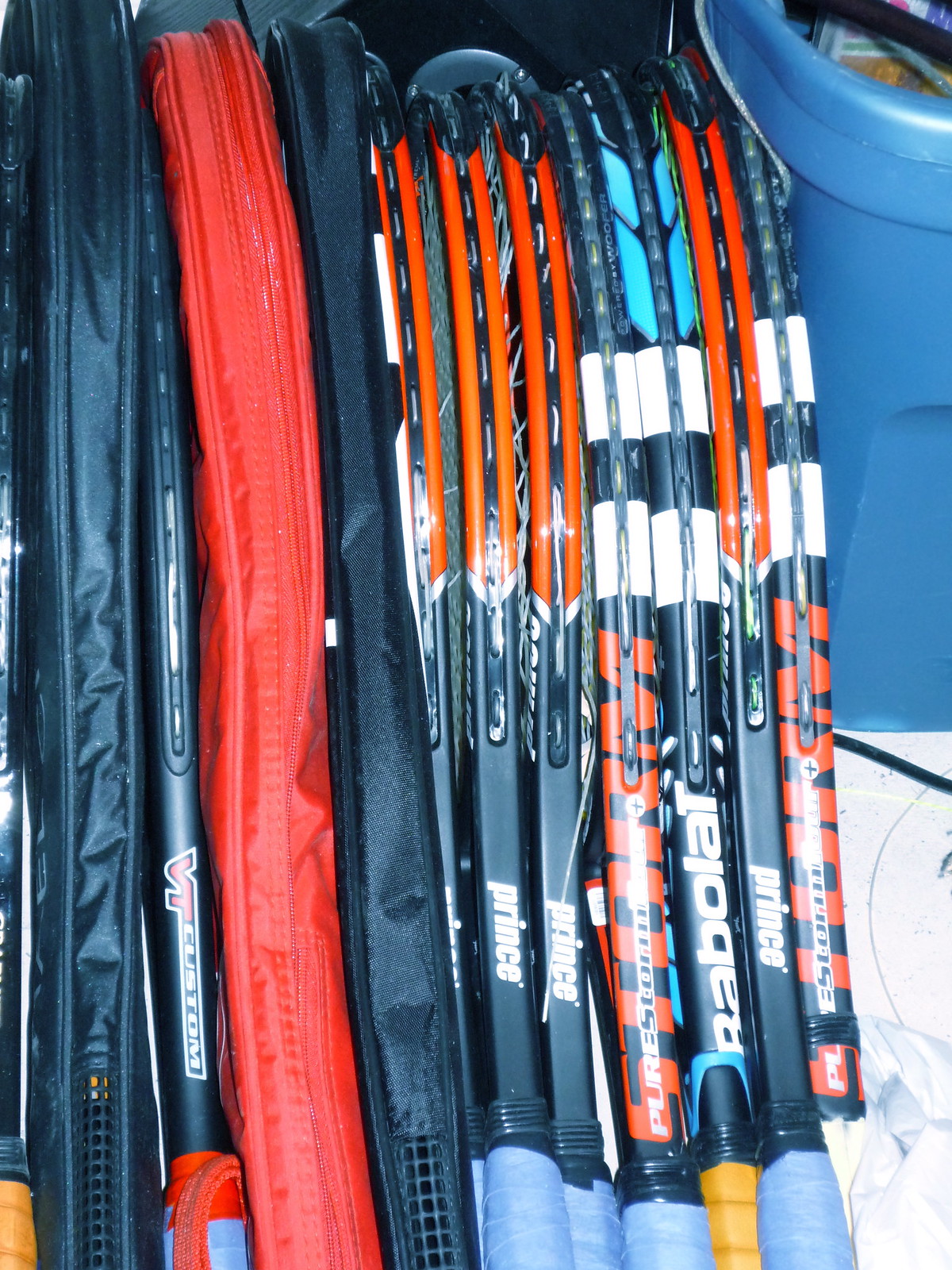This detailed photograph captures a close-up view of a vibrant array of tennis rackets displayed in a sporting goods store. The rackets are stacked side by side, with only the upper parts and mid-handles visible, creating a colorful and somewhat chaotic scene. Predominantly black, these rackets feature splashes of orange, light blue, red, and yellow. The display includes various recognizable brands, notably several Prince rackets and a few branded as DaViti Custom and Babelot. Some rackets are enclosed in protective cases—mostly black, with at least one red case—while others are displayed without covers, allowing intricate details and stitching on the frames to be seen. Toward the right side of the image is a large, blue plastic storage bin, suggesting an organized storage or a loading area. The handles mostly exhibit pale blue hues, contrasting against the different colored frames, making for a visually striking image of an enthusiast's or team's collection of tennis equipment.